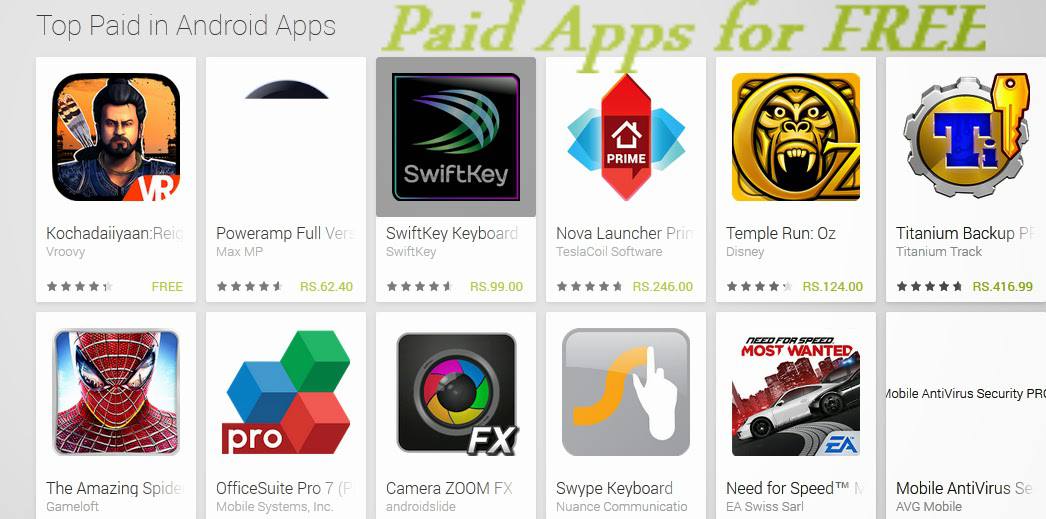The image depicts a collection of top-rated paid Android apps, accompanied by vibrant green text that reads "Paid Apps for Free." The assortment primarily features game applications. The first icon displays a bearded man equipped with a bow and arrow, labeled with "VR" and indicating it's available for free.

Other notable apps include:
- **SwiftKey Keyboard**: Developed by SwiftKey, normally priced at RS 99.00.
- **Temple Run: Oz**: An adventurous endless runner game.
- **Titanium Backup**: A robust backup utility tool.
- **Need for Speed: Most Wanted**: A thrilling car racing game.
- **Mobile Antivirus**: Security software to protect your device.
- **Swipe Keyboard**: An alternative typing tool.
- **Camera Zoom FX**: A powerful camera app for enhanced photography.
- **OfficeSuite Pro 7**: A professional office suite.
- **The Amazing Spider-Man**: Developed by Gameloft, featuring a red and blue Spider-Man avatar.

App icons are displayed in a typical format seen post-download and each app includes its price status—either free or discounted—and a corresponding star rating.